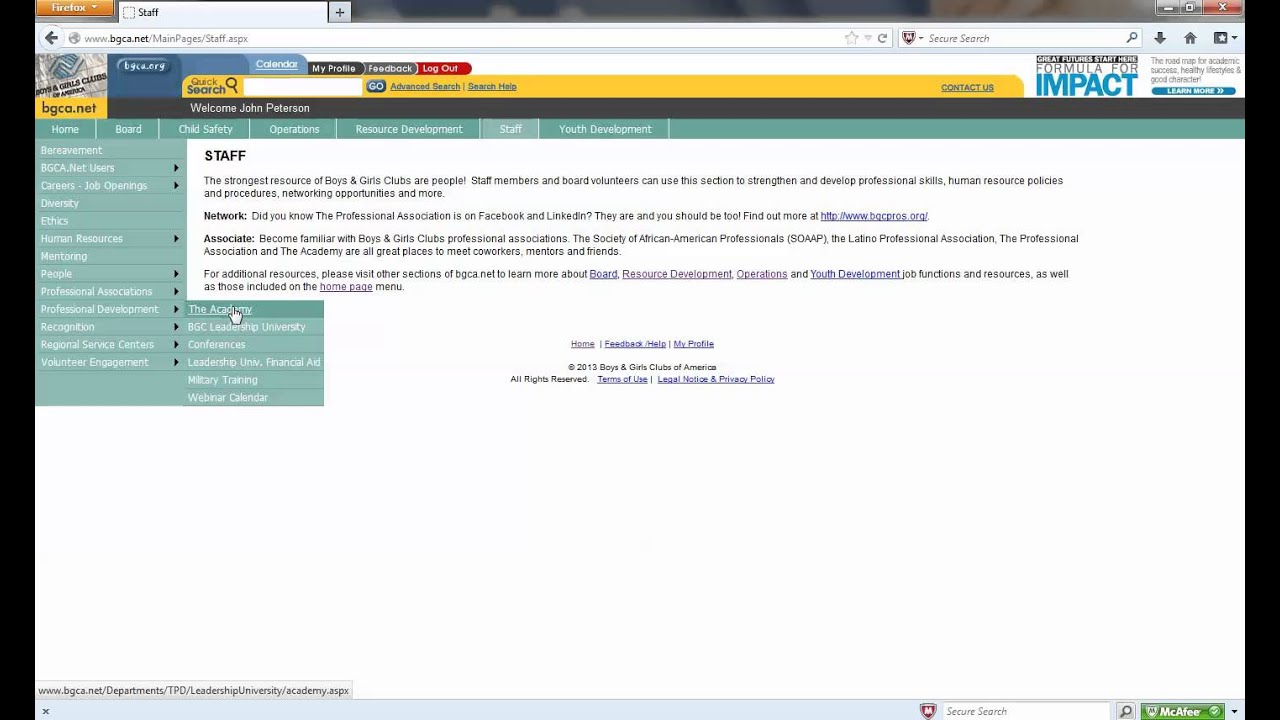Centered on the page, there is an informative section with a white background and prominent text conveying the key message: "Staff: The strongest resource of Boys and Girls Club is people." This section highlights how staff members and board volunteers can leverage this area to enhance their professional skills, human resource policies, procedures, networking opportunities, and more. It encourages engagement with the Professionals Association on Facebook and LinkedIn and directs users to bgcpro.org for more information. Additionally, it promotes familiarity with various professional associations such as the Boys and Girls Club Professional Association, the Society of African American Professionals (SOAPAP), and the Latino Professional Association. These groups serve as excellent platforms for networking, finding mentors, and making friends. For further resources, visitors are guided to explore bgca.net, where they can learn more about sports resource development, operations, youth development, job functions, and additional resources available on the homepage.

On the right side, the background changes to a vibrant green, listing essential site sections such as career job openings, diversity, ethics, human resources, mentoring, professional associations, professional development, recognition, regional services, volunteer engagement, academy, BGC, tenureship, university conferences, leadership university, financial aid, military training, and webinar calendar.

At the top of the page, a yellow section features a search bar with options for a quick search, advanced search, search help, and contact information. The top left corner prominently displays the website's URL, bgca.org.